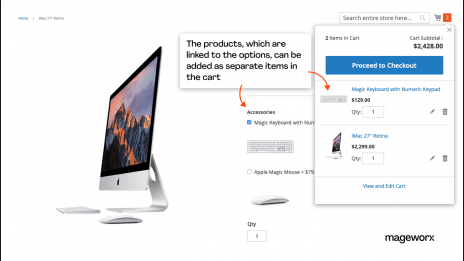This is a screenshot from an e-commerce website specializing in electronics. The image is slightly blurry with some text appearing small and hard to read. In the bottom right corner, there's a logo on a white background that reads "MAGEWORX" in black small caps. The left side of the image prominently features a white Mac desktop setup, complete with a keyboard and mouse, all Apple products. The computer screen displays a beautiful, snowy mountain range viewed from a high altitude.

To the right of the desktop, a text box with black text on a white backgroundstates, "The products which are linked to the options can be added as separate items in the cart." Nearby, an orange arrow points towards 'accessories,' and another orange arrow points towards the keyboard listed in the shopping cart. The accessories listed include the keyboard and the mouse, indicating that these are sold separately and do not come with the Mac desktop. The total price displayed for the Mac desktop, including the keyboard, is $2,428.